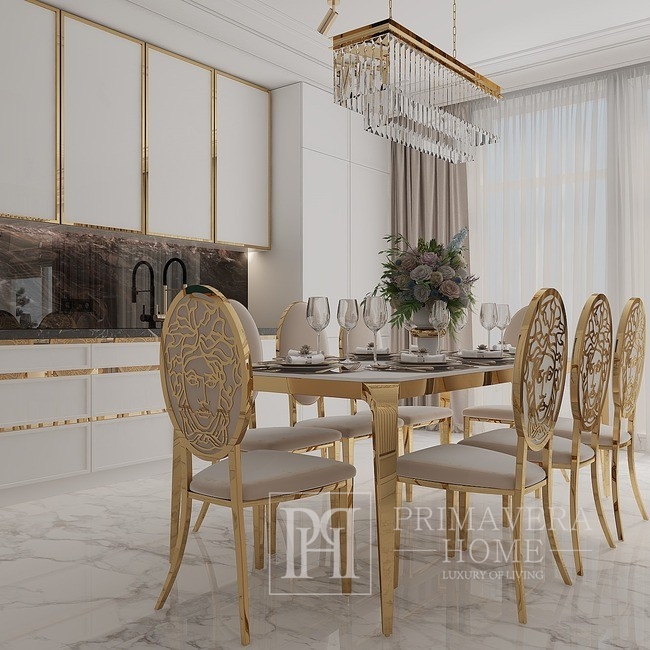This detailed color photograph, digitally enhanced and captured indoors under artificial light, showcases a luxurious dining area marked by elegant design elements. Central to the image is a gold metal table with a pristine white top, surrounded by eight gold chairs adorned with white cushions. Each chair features an intricate metalwork design on its back, depicting a face with flowing hair and a mustache. The floor is an exquisite white marble with subtle grey streaks, enhancing the room's opulence. 

The walls are lined with white cabinets trimmed in gold, adding to the luxurious motif. One side of the room features a counter with an elaborate faucet, suggesting a kitchen or dining setting in a sophisticated home. A gold and silver chandelier with reflective panels hangs above the table, casting shimmering light and reflecting the room's elegant surroundings.

On the right side, a window with a sheer curtain allows natural light to filter in. The table is set with fine plates, silverware, and a total of seven wine glasses, indicative of a formal dining arrangement. At the center of the table sits a striking bouquet in a white vase with gold trim, featuring blue and pink flowers with green stems. 

The image includes an added logo at the bottom center, displaying "Primavera Home Luxury of Living" within a square, where the “P”s face each other. The overall ambiance suggests a simple yet luxuriously styled apartment dining area.